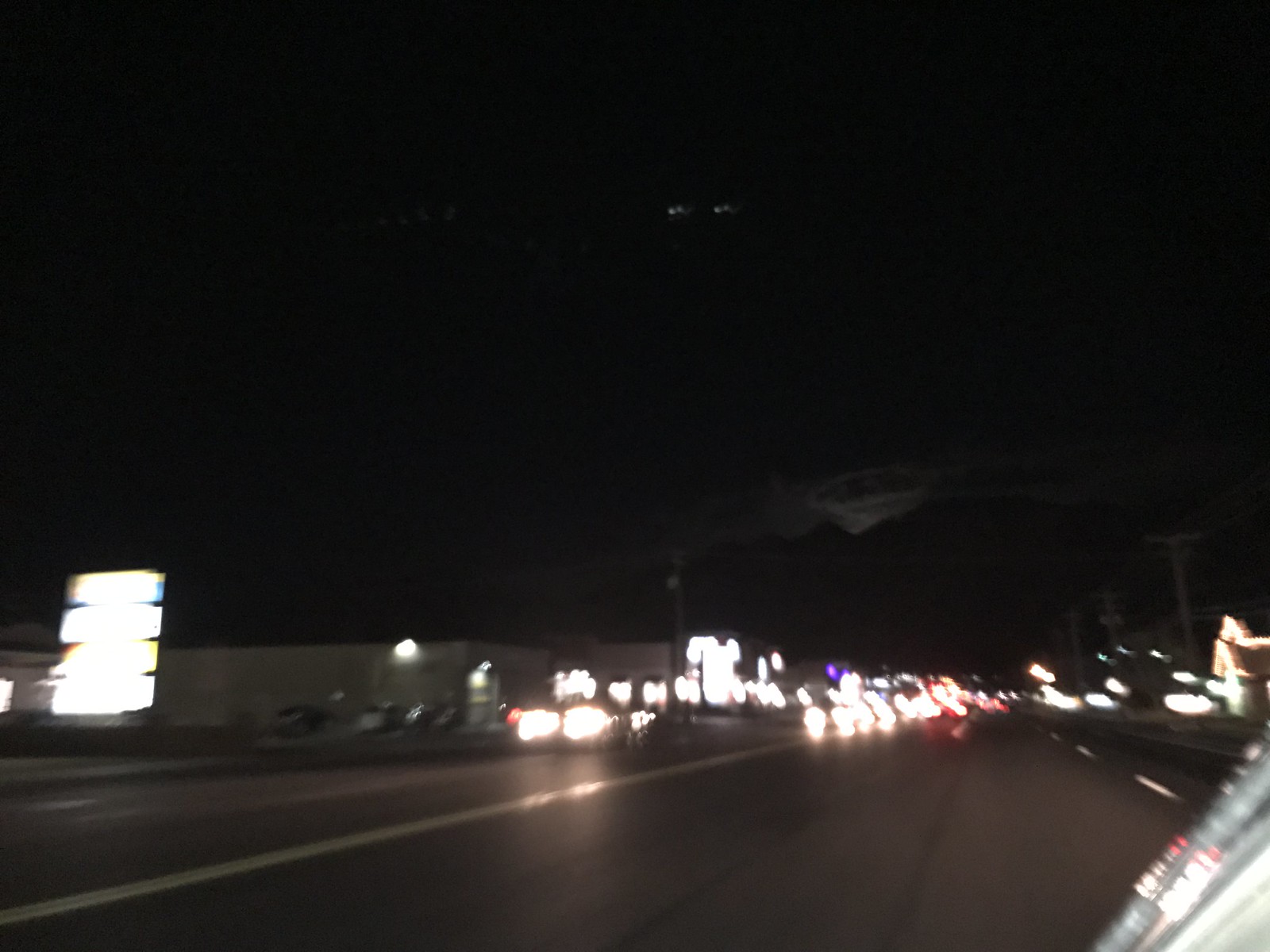The photograph captures a blurry nighttime scene taken from the side of a dark highway with multiple lanes. The sky above is black with faint, blurry clouds and secondary reflections from the camera lens. In the foreground, the asphalt road is visible, marked by white stripes dividing the lanes and double yellow lines on the left distinguishing oncoming traffic. Multiple cars with illuminated headlights drive towards the viewer, creating a stream of light against the dark setting. On the right side of the image, there are unlit street lights and overhead wiring. The left side reveals some illuminated structures, possibly a gas station and a couple of buildings or shops, while the far distance shows a few more buildings and electric poles. The entire image has a sense of motion, contributing to its overall blur.